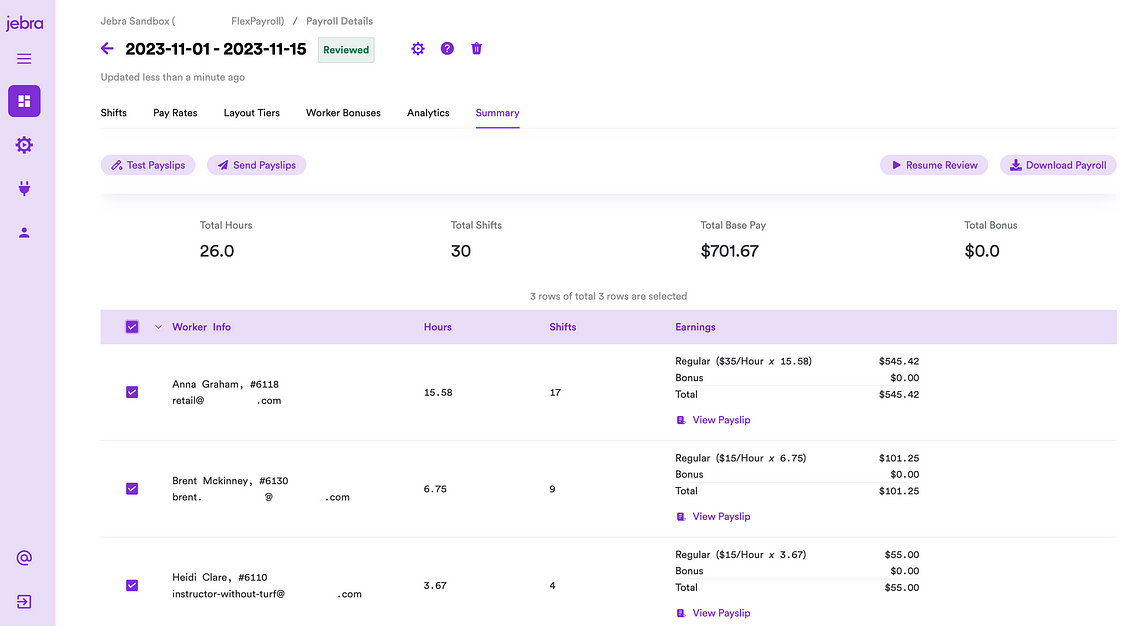The image primarily features a white background with a distinct lavender-colored rectangular box on the left-hand side that extends vertically. At the top of this lavender area, the text "JEBRA" is prominently displayed in dark purple, accompanied by three purple lines. Adjacent to the text, there is a purple square containing four small white squares and a purple-gray gear symbol. Below these elements, there is an icon that resembles a purple train and another representing a purple person.

Across the top portion of the image, it reads "Jefferson Box (Flex Payroll / Payroll Details)," with a purple arrow pointing to the left. Just below this, in black text, the date range "2023-11-01 to 2023-11-15" is visible. A green box with the word "Review" in dark green is also present.

Further down, several icons appear: a purple gear, a purple circle with a white question mark, and a purple trash can. There is an indication that the information was "Updated less than a minute ago."

Below this, you see headers in black text listing various categories: "Shifts," "Payrates," "Layout," "Tiers," "Worker Bonuses," and "Analytics." The section labeled "Summary" is underlined, and it provides detailed information on "Total Hours" (26.0) and "Total Shifts" (30). Additionally, it is noted that "three rows are selected."